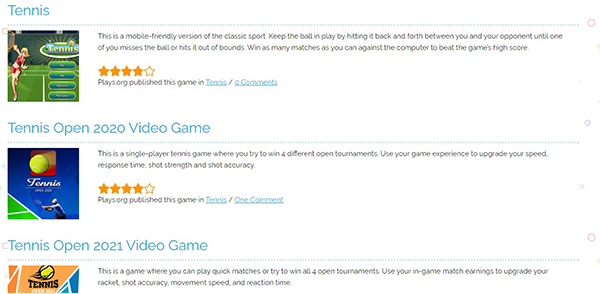This is an informational website dedicated to tennis. The top navigation bar prominently features the word "Tennis" and conveys its mobile-friendly nature with a clear emphasis. A primary image on the site shows a blonde woman dressed in red, poised on a grass court, ready to hit a tennis ball.

The site offers detailed insights into the classic sport, emphasizing that players aim to keep the ball in play by hitting it back and forth until one player misses or hits it out of bounds. The objective is to win as many matches as possible against the computer, striving to achieve the game's high score. This section has a rating of four out of five stars and includes links to terms and conditions that users can read for more information.

Additionally, the website features information about the "Tennis Open 2020" video game. This single-player game challenges players to win four different open tournaments. Gamers can use their experience points to upgrade various aspects such as speed, response time, shot strength, and shot accuracy. This game also boasts a four out of five gold star rating and is represented with a cover image of a male tennis player beside a large tennis ball under the bold title "Tennis."

The last section, though partially cut off, pertains to "Tennis Open 2021" video game. This game allows players to compete in quick matches or aim to win all four open tournaments. Players can use their in-game earnings to upgrade their racket, shot accuracy, movement speed, and reaction time. It includes a banner image prominently displaying the word "Tennis."